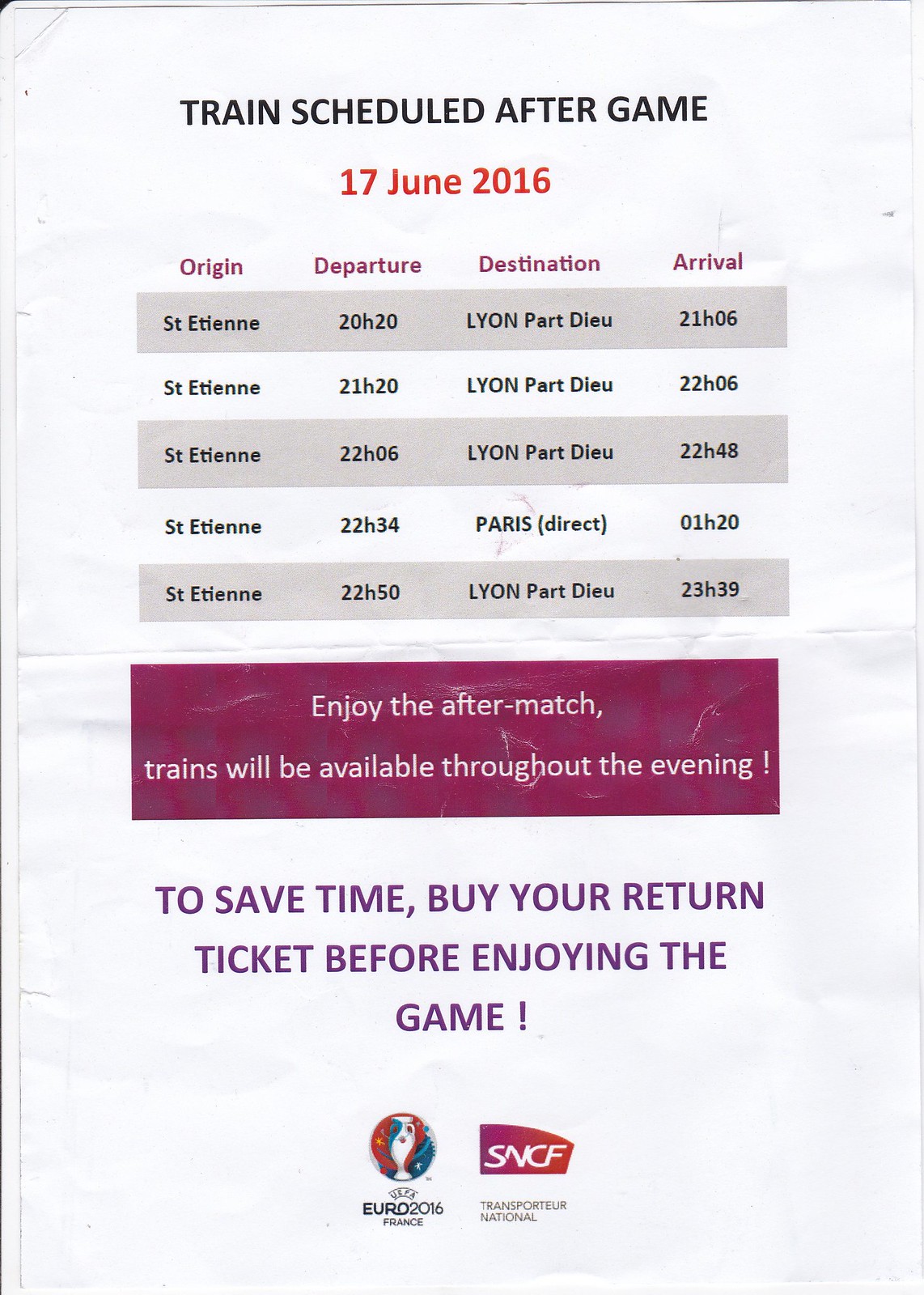The image depicts a slightly wrinkled, printed train schedule poster with a white background, seemingly photographed while hanging on a wall. At the top, in bold black capital letters, it reads "TRAIN SCHEDULED AFTER GAME." Directly below this, highlighted in red, is the date "17 June 2016." The schedule is organized into four columns with headings in a purplish color: Origin, Departure, Destination, and Arrival. All trains originate from Saint-Étienne, with five departure times listed as 20H20, 21H20, 22H06, 22H34, and 22H50. The destinations include Lyon-Part-Dieu for four trains and a direct route to Paris for one train. Corresponding arrival times are 21H06, 22H06, 22H48, 23H20, and 23H39, respectively. Below the schedule is a red box containing the white text "Enjoy the aftermatch. Trains will be available throughout the evening." Beneath the red box, in purple text, it advises, "To save time, buy a return ticket before enjoying the game." At the very bottom, the poster features two logos: one for SNCF Transporter Nationale and another for Euro 2016 France, which includes a graphic of a soccer ball.